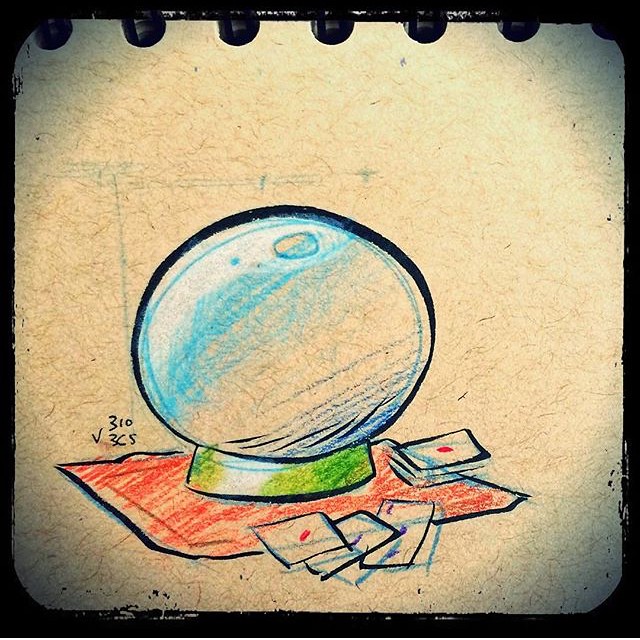The image displays a meticulously crafted drawing on a sketch pad. The artwork, rendered in black ink, is accentuated with vibrant crayon colors. Central to the piece is a crystal ball, exquisitely shaded in varying hues of blue—light blue, medium blue, and dark blue. The base of the crystal ball is colored a rich green, providing a solid foundation. This mystical object is placed atop a rectangular piece of paper, vividly colored in red, creating a striking contrast. Surrounding the crystal ball are several playing cards, intricately drawn and scattered around, adding an element of intrigue and mystery to the composition.